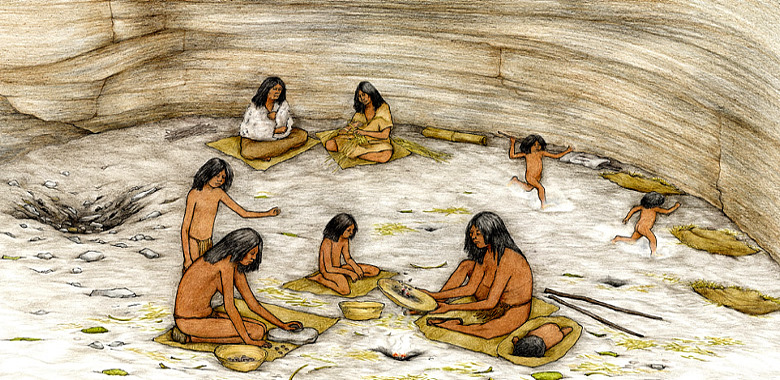This detailed illustration, made with colored pencils, depicts a scene from a pre-modern, possibly Mesoamerican civilization. The setting appears to be a large, cave-like structure with a curved rock or mud wall, creating an enclosed environment bathed in tans and golds. The inhabitants are indigenous people with mid-tone to dark brown skin and long black hair extending beyond their shoulders. 

Family groups are portrayed engaging in various activities. In the foreground, a woman, topless, is busy threshing grain next to an infant lying on a tan mat. Nearby, another woman grinds something on a flat stone, with a child in a loincloth standing behind her. There are also mats scattered around, green, yellow, and brown, used to protect them from the ground.

In the background to the left, there are two women sitting cross-legged on mats. One wears a white fur coat, and the other, dressed in a deerskin top, is weaving straw into more mats, evidenced by a rolled mat behind her. To the right, an open area reveals two naked young children gleefully running and playing, with one seemingly throwing something at the other. Additionally, another child kneels on a mat.

The floor is a mix of dirt and scattered rocks, featuring a rock pit—likely a fire pit—on the left side. Various objects such as spears and bowls lie on the ground, adding to the scene's authenticity. This richly detailed illustration captures a moment in the daily lives of this ancient community, emphasizing their activities, attire, and interactions within a protective, rock-walled enclosure.